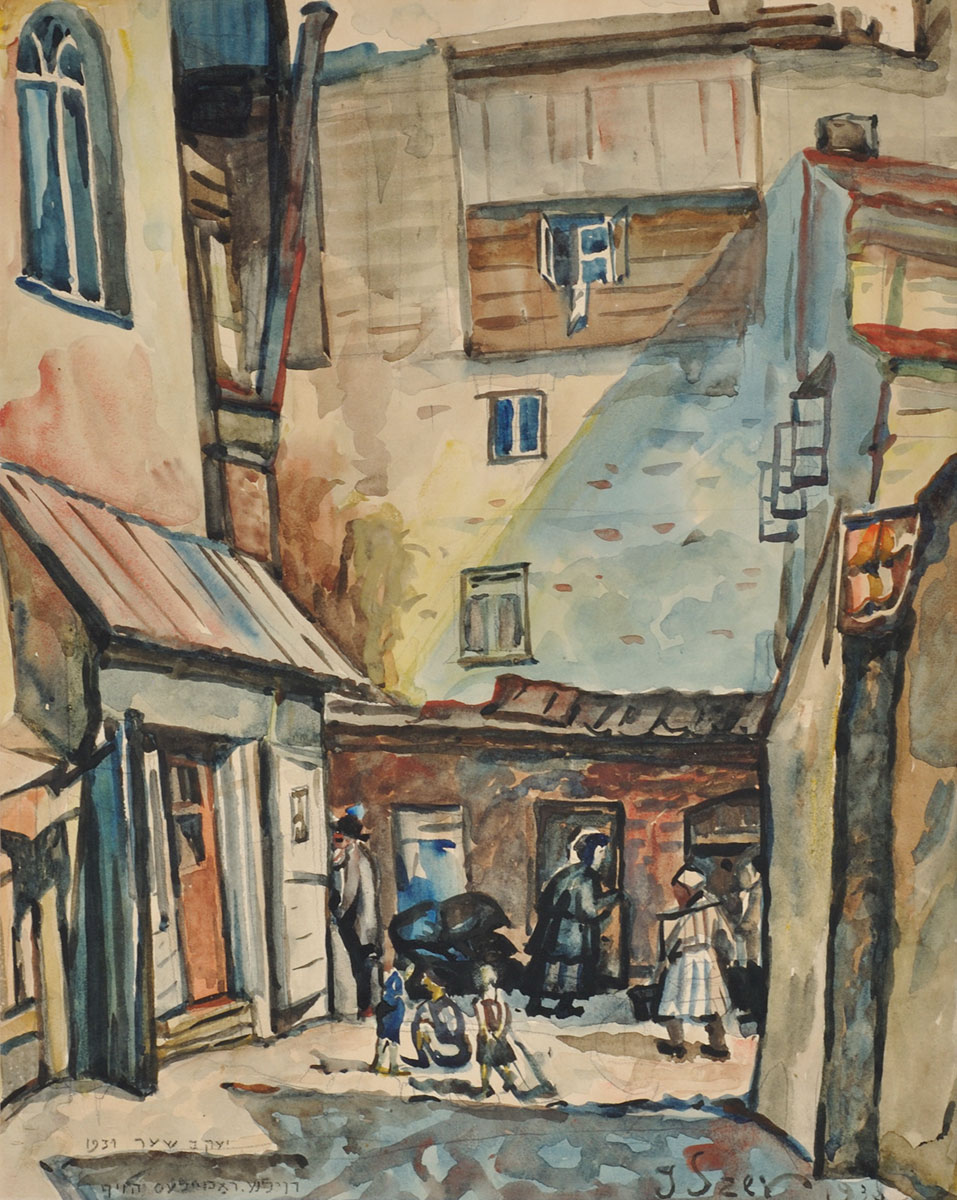The painting is a vertical watercolor depicting a quaint, historic town scene reminiscent of the late 1800s to early 1900s. The colors are primarily muted browns, blues, tans, and touches of red, lending a nostalgic feel to the artwork. The narrow walkway is flanked by older types of buildings, characterized by architectural features such as arched windows, dormers, and front doors. Notable structures include a curved arched window and a protruding dormer with a door on the far left, a house with four windows and another dormer in the center, and the side view of a house with open second-floor windows on the far right.

The scene is bustling with life; a woman is seen carrying water buckets on her shoulders, children play on the ground, and a man is walking into a store. The painting captures a lively street scape filled with approximately six people including both adults and children. Intriguingly, there is handwritten text in the bottom corners of the painting. On the right side, it reads "G.S. Sear, 1936," while on the left, it is inscribed "J. Scene, 1933," adding a layer of historical context and artist personalization to the piece.